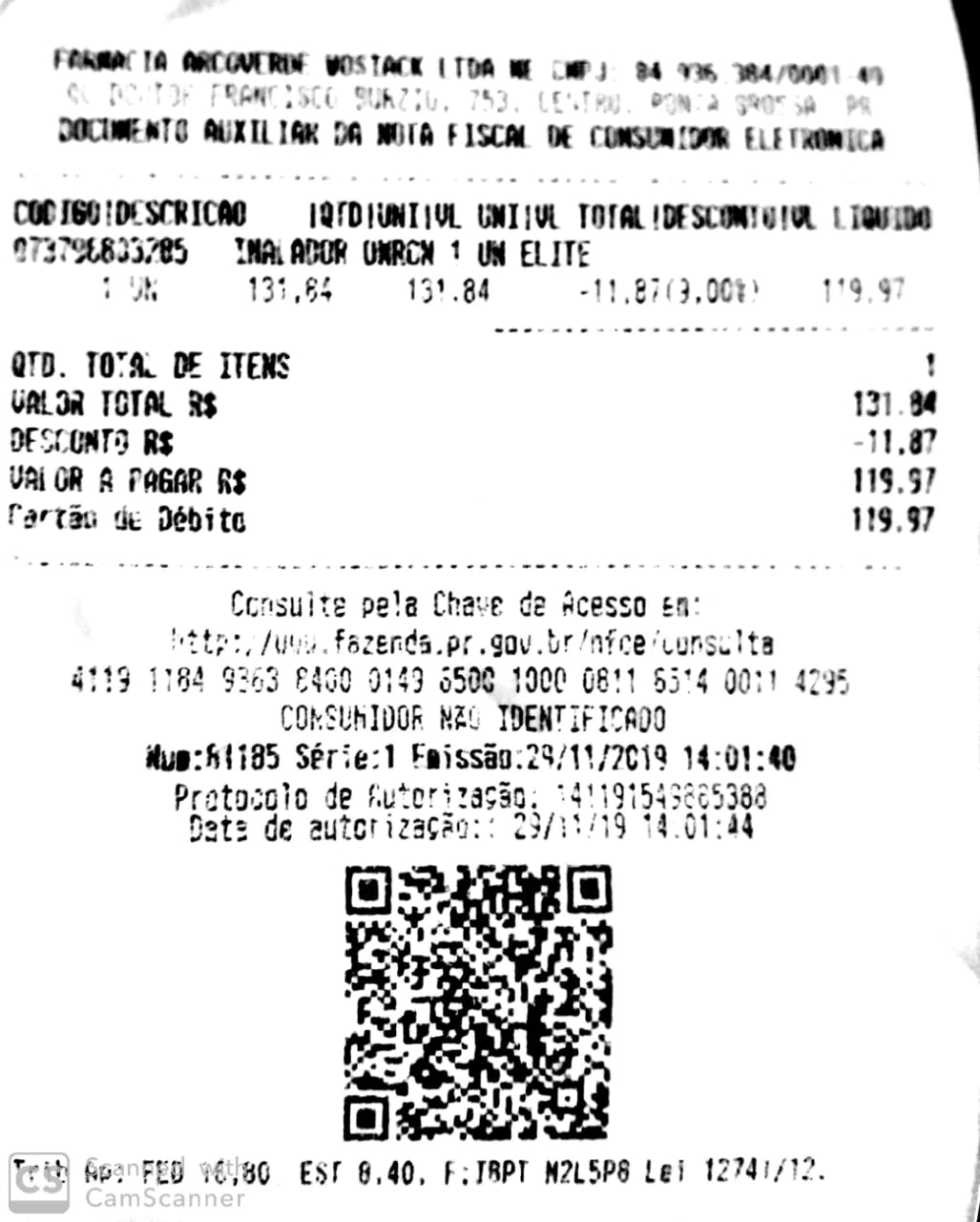This image is a close-up, black-and-white photograph of a receipt. The receipt dominates the frame, albeit with a small portion in the upper right-hand corner where a sliver of a dark background is visible. In the lower-left corner, the watermark "CAM scanner" is present alongside a square logo featuring "CS." The receipt showcases a QR code at its base and records a total amount of $119.97. Certain text elements on the receipt appear darker and more pronounced, while other parts are faint and difficult to read, adding a degree of complexity to deciphering its full details.